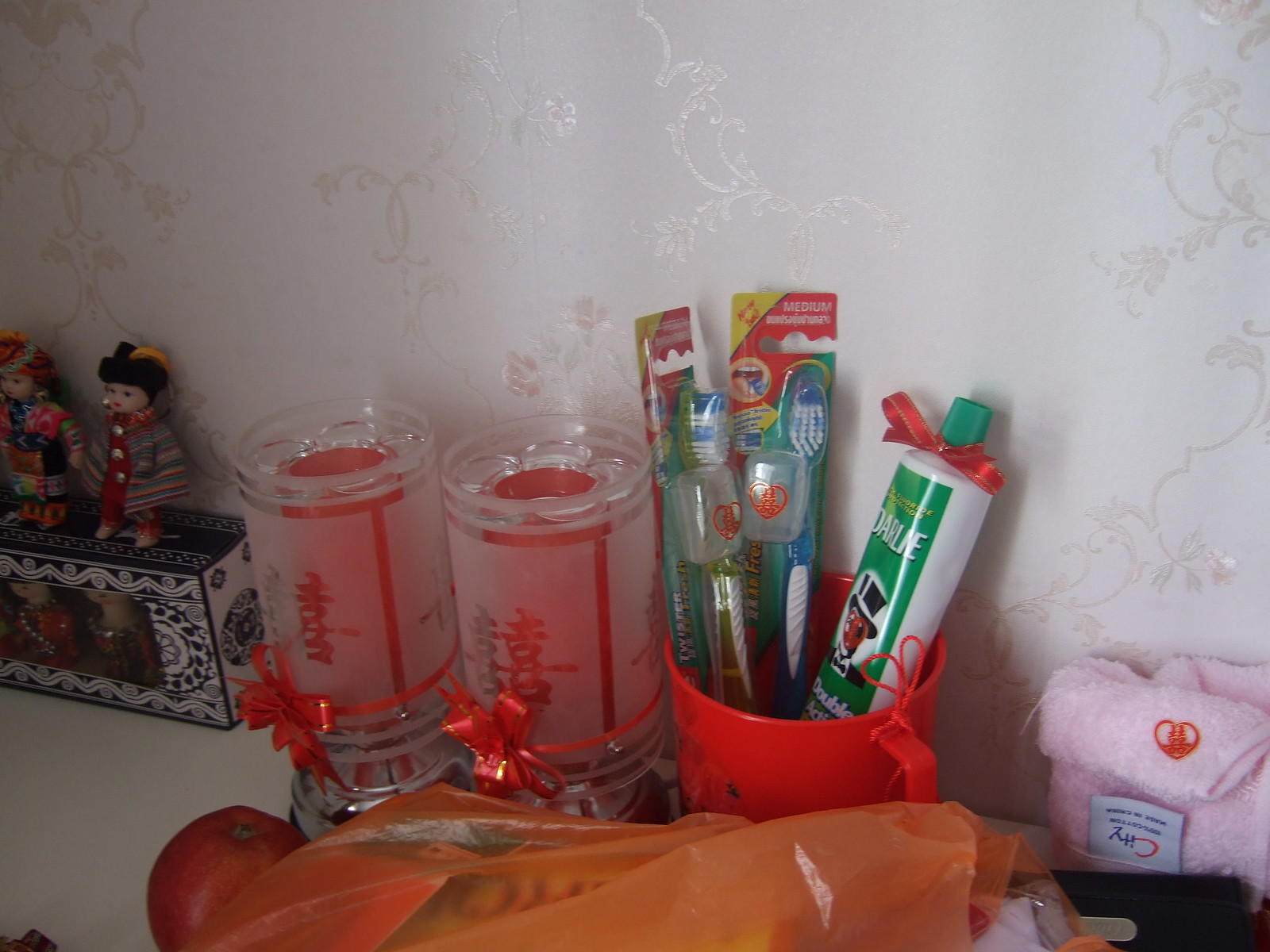The image captures the interior of a home adorned with a white wallpaper embellished with a shiny, golden floral pattern. At the very center bottom, an orange bag partially filled with unspecified items stands out. To its right, a red cup with a handle holds two brand new toothbrushes, fully packaged and equipped with toothbrush head covers; one package is legibly marked "medium." A white and green toothpaste tube wrapped with a red ribbon is also placed inside the cup. Adjacent to the cup on the right, a pink towel rests, while on the left, two glass candle holders with Asian lettering and red bows contain red candles. Further left, a set of small Asian dolls, one male and one female, wearing detailed knitted clothes, stand on a box that appears to contain more figurines. An apple is positioned near the cup, contributing to the diverse collection of items displayed.